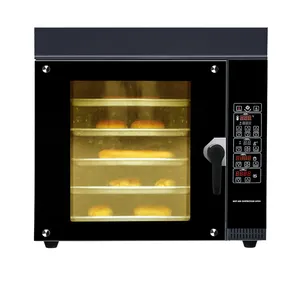This image depicts a square-shaped, black oven, distinctly set against a white background, emphasizing a clean, product photography aesthetic. The oven features a transparent glass door, allowing a clear view of its interior, which is fitted with five rows of chrome-colored aluminum pans stacked one above the other. Each pan is adorned with different pastries or breads, showcasing the appliance's baking capabilities. The door, accented with a black handle located in the center-right, is bordered by four silver screws at each corner, adding a sturdy, utilitarian detail. To the right of the door, a vertical control panel houses about five rows of buttons, enabling precise selection of baking settings. The top part of the oven contrasts slightly with a gray hue, demarcated by a dividing line from the rest of the unit. Short black legs at the base give the oven stability, while the overall setting suggests a high-quality, detail-oriented promotional portrayal, reinforcing the oven’s functionality and elegant design.